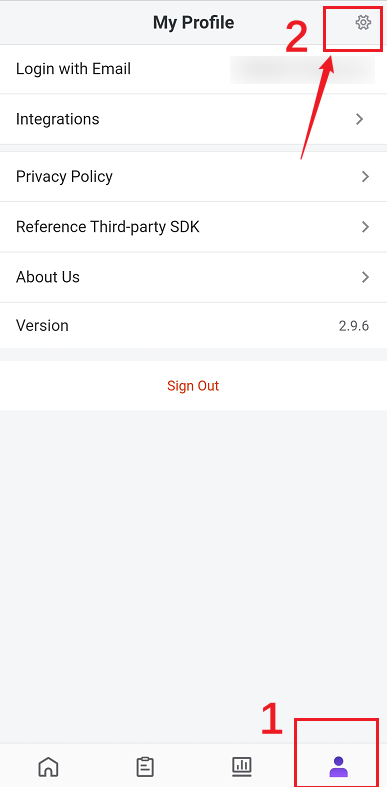This image appears to be a detailed screenshot taken on a smartphone, displayed in a vertical orientation. At the top, there is a header labeled "My Profile" accompanied by a bolt symbol in the upper right corner. The bolt symbol is highlighted with a red square and an upward-pointing red arrow, annotated with the number "2" in red on the left side. Below the header, a list of options is presented in black text, which includes "Login with Email," "Integrations," "Privacy Policy," "Reference," "Third-Party SDK," "About Us," and "Version." At the very bottom center of the screen, the text "Sign Out" is displayed in red, followed by an empty gray box beneath it. In the bottom right corner, there is another red square surrounding a purple person icon, marked with the number "1" in the top left corner of the square. The red boxes and their associated numbers and symbols seem to be connected, possibly indicating linked or sequential elements within the app's interface.